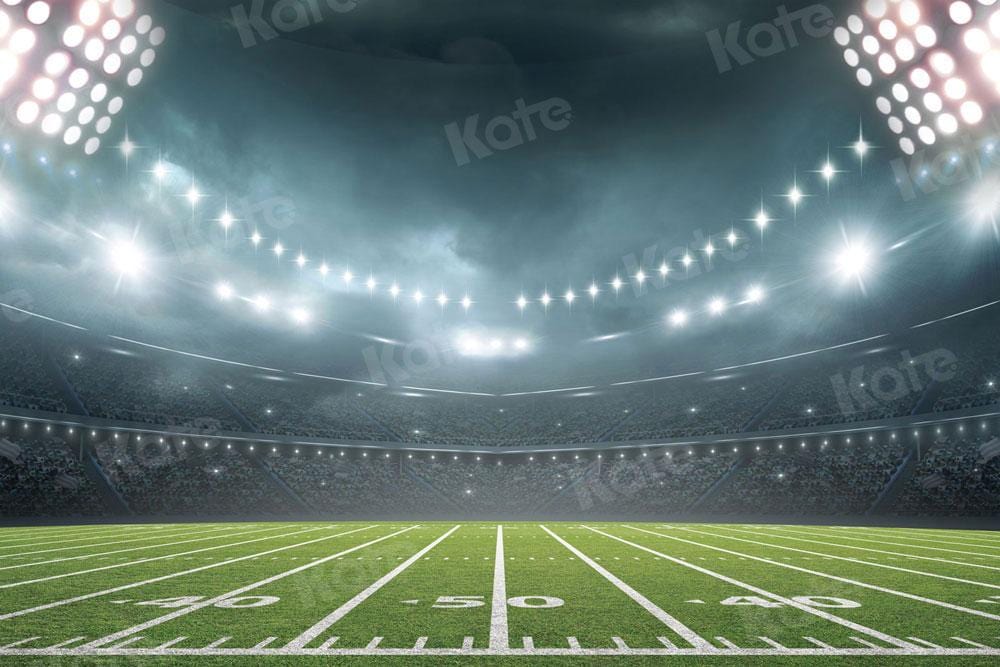The image depicts a symmetrical football field inside a stadium, prominently marked by a green turf with white lines and ticks, including a central 50-yard line flanked by 40-yard lines. The field occupies the bottom 20% of the image, with detailed white markings and evenly spaced ticks along the sidelines. Surrounding the field are two levels of stands, appearing full of people and illuminated by extensive lighting situated at the top left and right corners of the image. The stadium, which seems to be open-air judging by the foggy or smoky atmosphere, showcases symmetry along an axis extending from the 50-yard line. Additionally, the word "KATE," designed in a copy-light style, is watermarking the entire image.